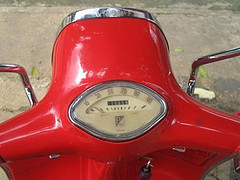A bright cherry-red Vespa scooter takes center stage in this photograph, its gleaming chrome accents capturing the light and adding a touch of elegance to its classic design. The headlight, encased in shiny chrome, stands prominently at the front, while chrome bars rise up the sides, reflecting the vivid red body. The speedometer, uniquely shaped with a rounded top narrowing to a point at the bottom, features a light brown background with clearly visible numbers and an odometer. The backdrop suggests a vintage European street, possibly in Paris or Italy, with its worn, brown-hued cobblestones and an overall old-world charm. Subtle details, like specks of moss and scattered leaves, contribute to the serene and timeless ambiance of the scene.